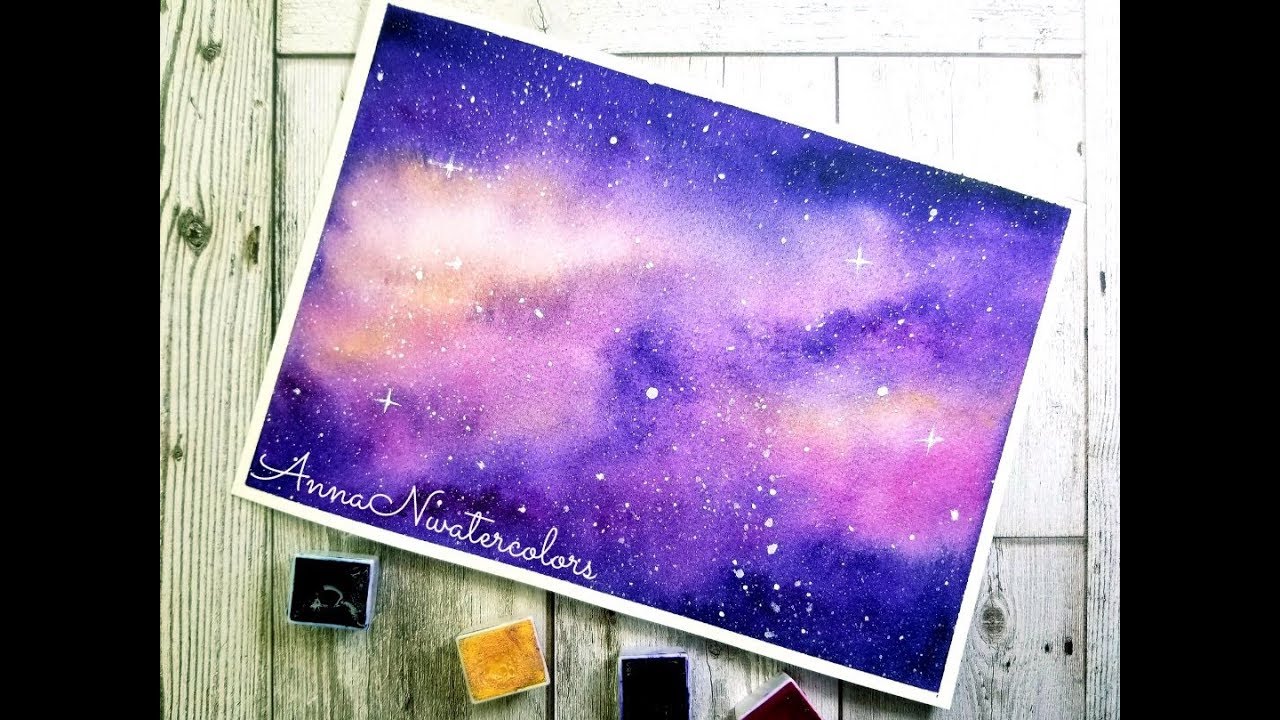This image portrays a captivating night sky scene, bordered by a black and white wooden surface. The night sky is painted in rich shades of blue, purple, and pink, with a sparkling array of stars and wisps of white clouds. The central feature of the painting includes soft pink and tan clouds stretching from end to end, adding a dreamy quality. At the bottom of the painting, it is signed "Anna in watercolors," indicating the artist's name and medium. The image also features a couple of square-shaped stamps in black, yellow, and rust colors, placed at the bottom. Both the painting and the stamps rest on a wooden paneled surface, accentuating the artwork's rustic charm.